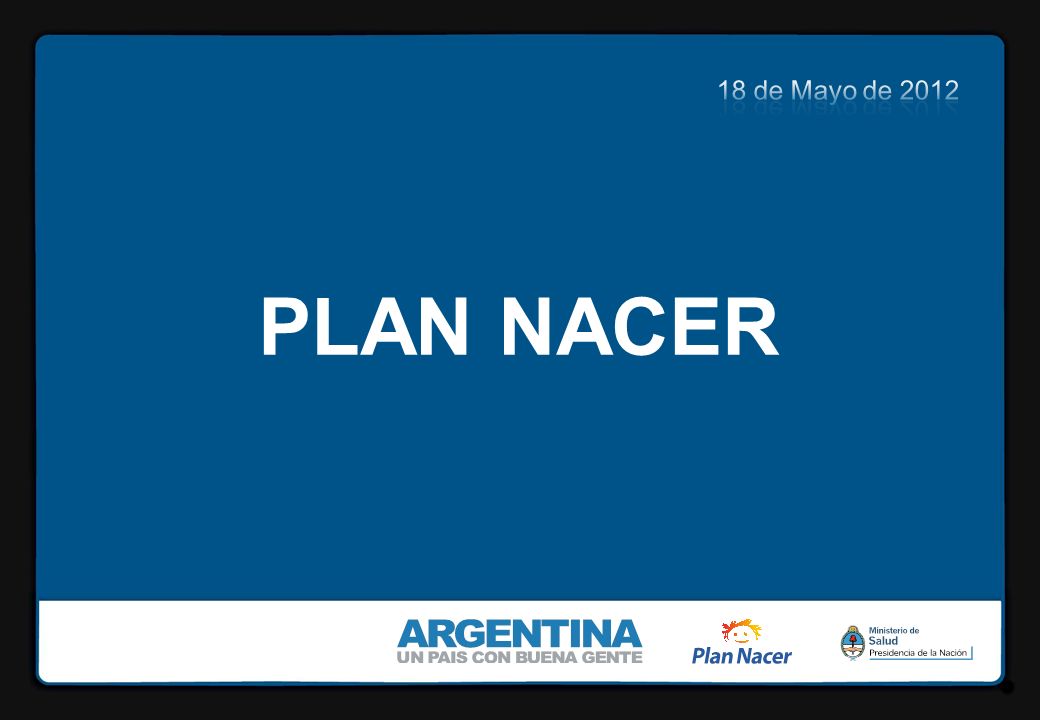The image appears to be an Argentine poster or flyer detailing an event or initiative dated May 18, 2012. It features a black background framing a darker blue rectangle with rounded corners, overlaying a smaller white rectangle at the bottom. In the top-right corner of the blue rectangle, the date is displayed in white text: "18 de Mayo de 2012." Dominating the center, also in white, are the words "PLAN NACER," written in all caps. 

Below the blue rectangle, in the white section, "Argentina" is prominently written in blue, and to its right, in gray, the phrase "Un País con Buena Gente" can be seen. Additionally, the blue-tinted logo features a cartoony child's face above the phrase "Plan Nacer" in gray text. Further to the bottom right, the text "Ministerio de Salud Presidencia de la Nación" is printed, indicating the involvement of Argentina's Ministry of Health. The composition of the text and logos suggests an official and promotional nature, emphasizing national health and community engagement.